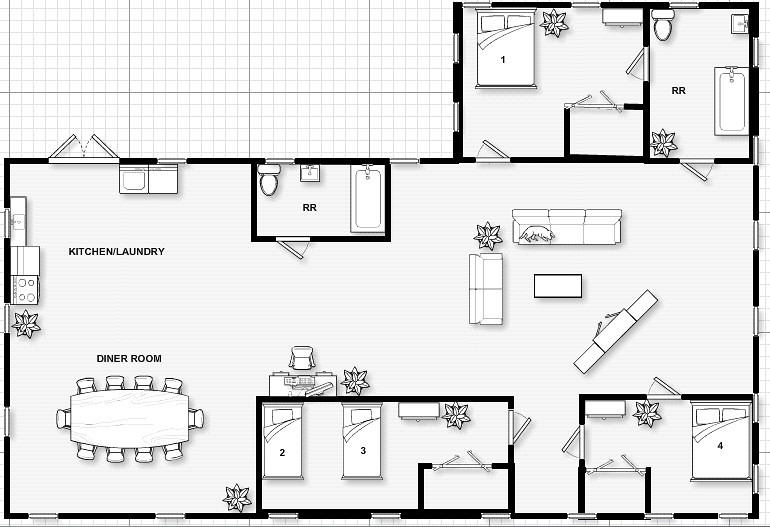This is a detailed top-down floor plan created using a computer program, clearly evident by its design on a computer-generated grid paper assuring precise measurements and placements. The primary layout depicts a mostly rectangular living space with an additional smaller extension at the rear of the house.

The living space, comprising about two-thirds of the bottom portion of the image, is organized into several clearly defined areas. At the top section of this main rectangle, you find the kitchen and laundry area. Directly beneath this, a dining room is situated, indicating an open-concept design that seamlessly integrates the kitchen and dining spaces.

Moving further along, there is a restroom positioned as a public facility for residents and guests. Across from this restroom is a bedroom. The entire layout features an open plan, ensuring a flow from the kitchen and dining room into a larger hall, which then leads into the living room. 

From the living room, there is a hallway that reconnects to the previously mentioned bedroom and proceeds to another smaller bedroom located to its right. The described extension off the primary rectangle includes additional rooms: another bedroom and a bathroom, providing extra private living spaces.

The meticulous design of this floor plan accentuates functionality and ease of movement, ideal for accommodating family life and entertaining guests.